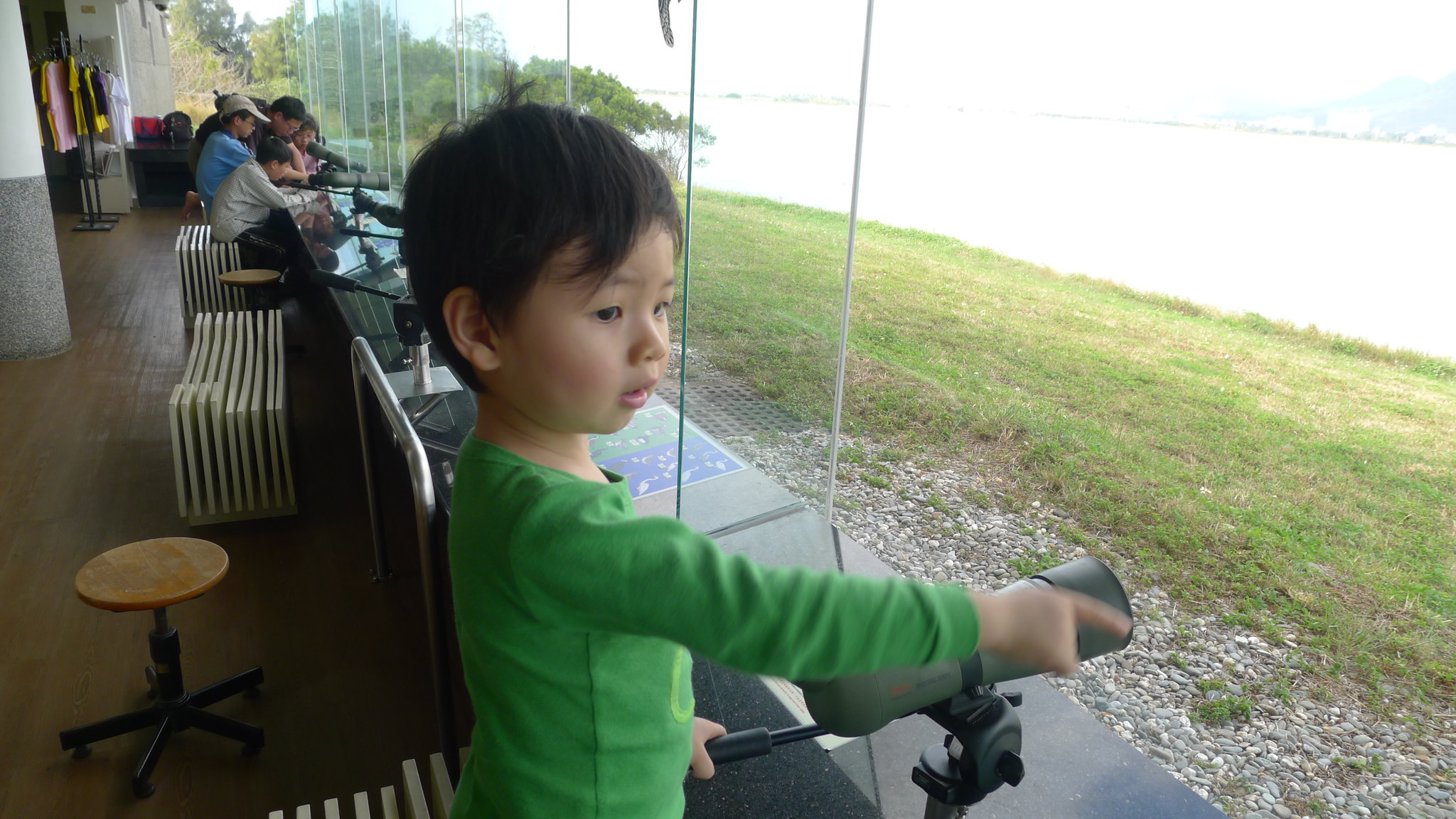The image showcases a charming scene at what appears to be a tourist attraction or observatory with a focus on bird watching or similar activities. A large, modern building with a glass wall forms the backdrop, creating an open, airy feel while still being an enclosed space. Inside, there are wooden chairs with unique, stacked designs and doctor-style rolling stools, all neatly arranged in symmetrical booths separated by glass partitions.

The building is situated next to a body of water, likely a lake, with a grassy patch and gravel area in between. The lake is on the right side of the image, partially washed out by sunlight, while the building is on the left. In the foreground, a young boy, around three to five years old, with shaggy black hair and wearing a long-sleeved green shirt, captures attention. He has his left hand on the handle of a mounted viewing device resembling binoculars or a telescope. He points off to the side with a slightly confused but cute expression, seemingly curious about something in the distance.

In the background, several people are using similar viewing devices attached to tables, possibly observing a landmark or wildlife across the lake. The scene combines elements of curiosity, exploration, and leisure, making it a compelling and heartwarming snapshot of human interaction with nature.